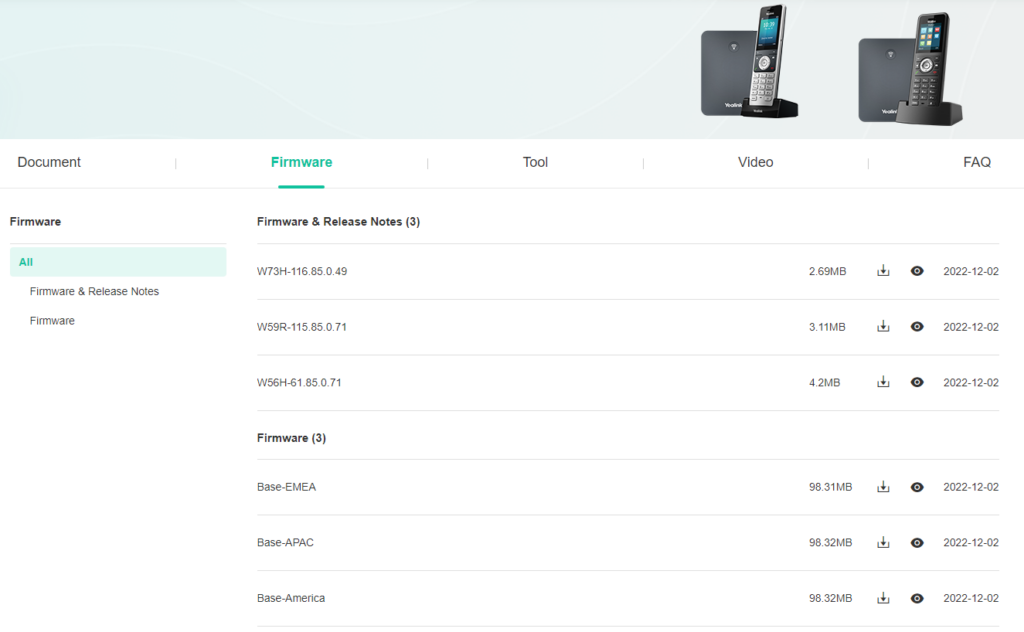In the top right corner of the image, there are two cell phones. One of them is entirely black featuring a screen filled with various icons, and it appears to be placed on a stand, charger port, or similar supporting device. The background shows a repeated pattern of this supporting device. The other phone is also black but has a touch of silver around the number pad area.

Below the phones, from left to right, there are several labeled sections: "Document," "Firmware," "Tools," "Videos," and "FAQs." Further down, there is a section titled "Firmware" followed by another labeled "Release Notes." Listed within these sections are firmware updates with their respective details.

One of the firmware listings is:
- W7-3H-116.85.0.49, 2.69 MB, with options to download (symbolized by a download button) or view more details (indicated by an eye icon). The date of this update is 2022-12-2.

Another firmware listing is:
- W59R-115.85.0.71, 3.11 MB, also with corresponding download and eye icons, dated similarly.

Each entry in the firmware section follows this pattern, providing a standardized way to access information and updates.